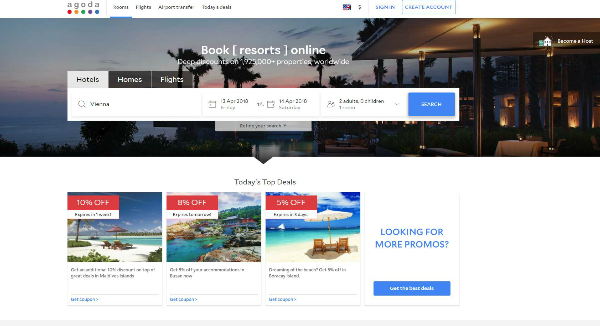This is an image of a web page from the travel booking website Agoda. The Agoda logo, featuring lowercase, gray letters "a-g-o-d-a" on a white background, is prominently displayed at the top. Below each letter, there are small, vibrant circles in red, orange, green, black, and blue. To the right of the logo, various navigation options are listed, including what appears to be "Lessons," "Flights," "Airport Transfer," and "Today's Deals." There are also buttons for signing in or creating an account.

Beneath this header, the page showcases a wide rectangular image of a patio dining setup at an upscale resort. The scene is set at night, possibly overlooking the ocean, and features beautiful scenery with palm trees in the background. The dining area is adorned with candles, adding a warm glow to the setting. Tables, covered with crisp white tablecloths, are arranged neatly in the patio area.

Overlaid on this scenic image, in white text at the top, are the words "Book [Resorts] Online." Below this text, a white search box is provided for users to enter their details and initiate a search.